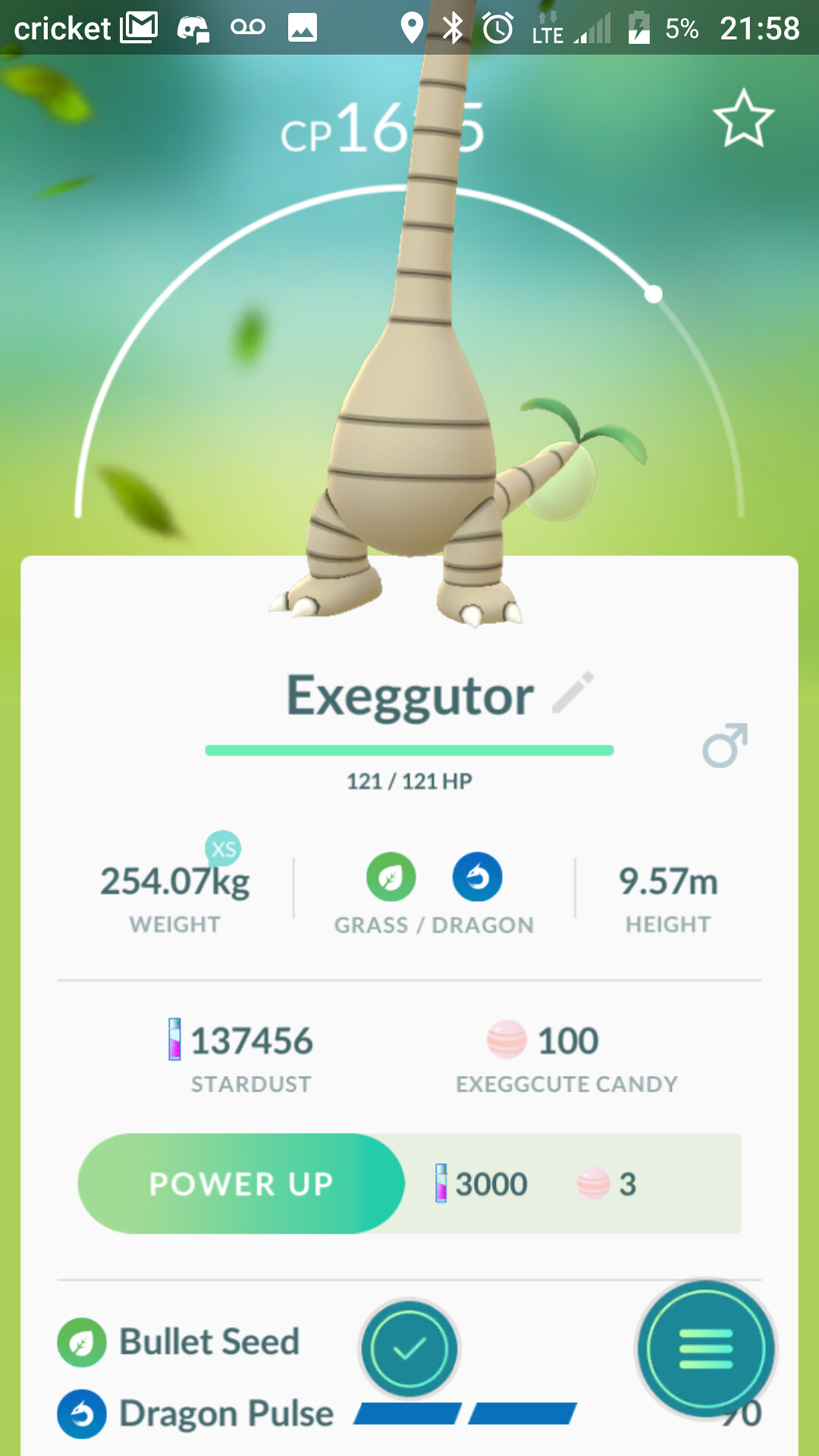This detailed screenshot from a phone displays elements from a mobile game interface. At the very top of the screenshot, against a green background with a darker green border, the word "Cricket" is prominently displayed in white. Adjacent to this is a letter "M". Moving towards the center, various icons indicate the phone's status, including battery life, which is critically low at 5%. The current time, shown to the right, is 21:58.

The remainder of the screenshot includes a blue and green background featuring a vibrant illustration of a unique animal. This creature has large white feet and a long neck reminiscent of a giraffe's, which extends upward to the top of the screenshot. The body of the creature is rounded, white, and adorned with brown stripes. Extending from its right side is a tail that features green sprouts.

Below the illustration, the word "Exeggutor" is prominently displayed, identifying the creature. Under this, a blue line serves as a divider. To the left of this line, various attributes of Exeggutor are listed: its weight of 254.7 kilograms, its types denoted as "Grass" (green) and "Dragon" (blue), and its height of 9.57 meters. Additional game-specific metrics include "Stardust: 137,456" and "100 Exeggutor Candy."

Towards the bottom of the screenshot, a green button with white lettering reads "Power Up". Next to it, a white background with dark letters reads "3000-3". The lowest section features move sets with symbols indicating the creature's abilities: a green circle with "Bullet Seed" and a blue circle with "Dragon Pulse." Under these headings, two check marks confirm selections. Additionally, a green circle with a white check mark and another green circle with three horizontal bars are visible at the lower right, all culminating to compile this in-depth overview of the game's interface.